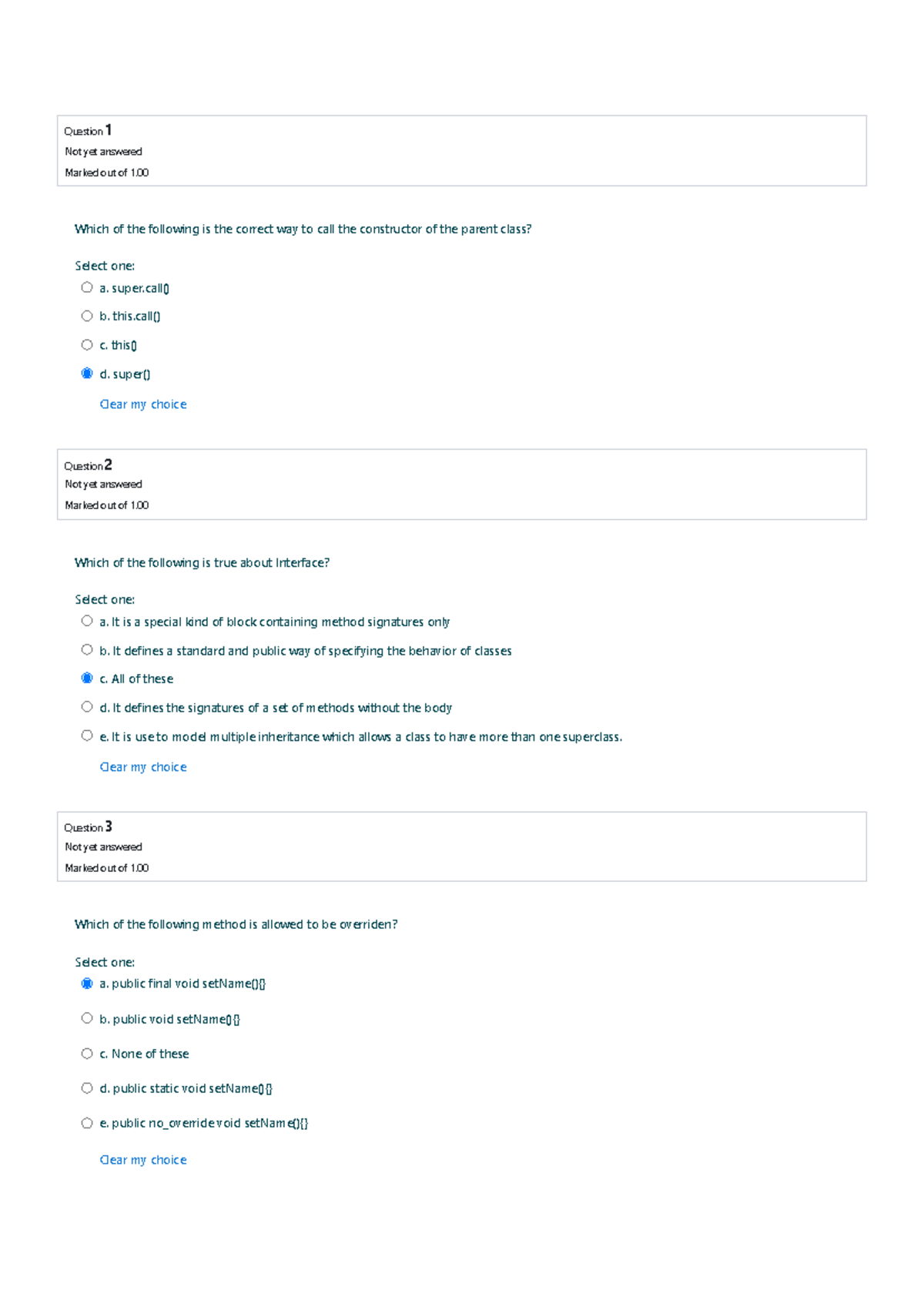Here's a cleaned-up and detailed caption for the described screenshot:

---

This image depicts a screenshot of an online quiz, displaying three multiple-choice questions related to programming concepts. No specific type of quiz is indicated.

1. **Question 1:** 
   - **Status:** Not yet answered, marked out of 1.00.
   - **Question:** "Which of the following is the correct way to call the constructor of the parent class? Select 1."
   - **Options:**
     - **A:** `super.call()`
     - **B:** `this.call()`
     - **C:** `this()`
     - **D:** `super()`
   - **Additional Detail:** A blue text option that says, "Clear my choice."

2. **Question 2:** 
   - **Status:** Not yet answered.
   - **Question:** "Which of the following is true about interface? Select 1."
   - **Options:**
     - **A:** "It is a special kind of block containing method signatures only."
     - **B:** "It defines a standard and public way of specifying the behavior of classes."
     - **C:** "All of these."
     - **D:** "It defines the signatures of a set of methods without the body."
     - **E:** "It is used to model multiple inheritance, which allows a class to have more than one superclass."

3. **Question 3:** 
   - **Question:** "Which of the following method is allowed to be overwritten?"
   - **Options:**
     - **A:** `public void setName()`
     - **B:** `public void setName()`
     - **C:** "None of these."
     - **D:** `public static void setName()`
     - **E:** `public no_override void setName()`

Each question requires the selection of one correct answer from the provided options.

---